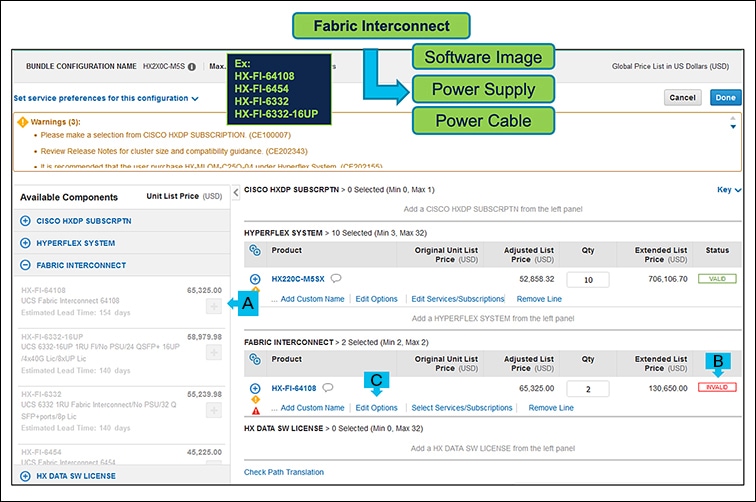This infographic outlines a purchasing guide for various Cisco products, detailing configuration specifics and associated pricing. It features a prominent black outline around a white block titled "Fabric Interconnect" in navy blue, set against a green rectangle. A blue arrow directs the viewer downwards and then to the right, pointing towards the "Power Supply" section. Above this, text reads: "Software Image" and "Power Cable."

The infographic references a bundle configuration named "HX2XOCM5S," with instructions to set surface preferences for the configuration. Readers are prompted to select from the "CISCO HXDP Subscription" and are advised to review release notes for cluster size and compatibility guidance.

Below this, an "Available Components Unit List in USD" section is detailed, listing "Cisco HXDP Subscription," "HyperFlex System," and "Fabric Interconnect." The "Fabric Interconnect" section is expanded, with a highlighted "A" in a blue box leading to grayed-out text.

On the right, the "HyperFlex System HX220CM5SX" is listed with an estimated list price of $706,106.70 for a quantity of 10 units, each priced at $52,858.32. Similarly, the "Fabric Interconnect FXFI64108" is priced at $65,325 per unit with a quantity of 2, totaling $130,650. This item is marked with a red "Invalid" indicator and has a "C" next to an "Edit Options" prompt.